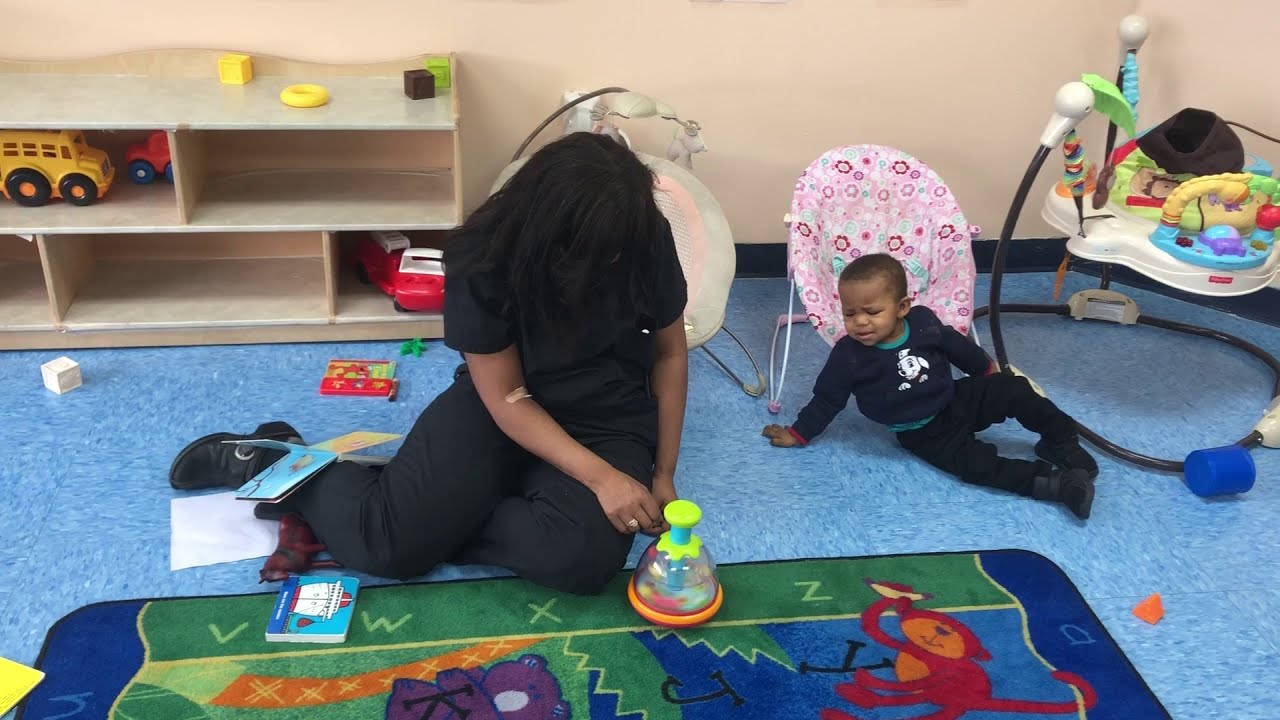In an indoor setting resembling a nursery or pre-kindergarten room with tan walls, a small boy in a navy blue sweater featuring an image of a dog, light blue t-shirt underneath, black pants, and black shoes sits on a blue linoleum floor. The boy, with short black hair, appears to be fussing, his face crinkled in displeasure as he leans on one hand, curving towards a female adult beside him. The woman, seated on the floor in black attire and black shoes, has her dark hair covering her face, obscuring it entirely as she plays with a toy using both hands. A Band-Aid is visible on her elbow. Scattered around them are colorful toys, including a red, blue, and green playmat depicting cartoon characters, pink and flowered play seats, as well as a white, purple, yellow, and blue rocker. The floor is dotted with various other toys, including small cycles, chairs, and books, adding to the lively, playful atmosphere of the room.